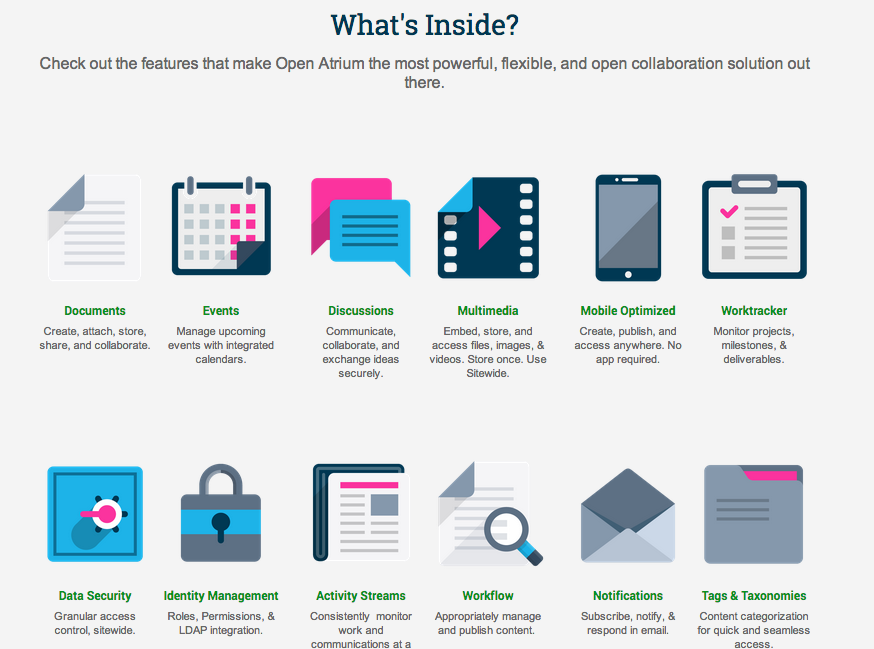On this page, a comprehensive overview of Open Atrium's features is presented in a clean and organized manner. At the top, the heading "What's Inside?" is displayed in a subtle grey font, creating a sense of curiosity and introduction.

Directly below this heading, the following phrase is displayed in grey font: "Check out the features that make Open Atrium the most powerful, flexible, and open collaboration solution out there."

Below this introductory text, there are two rows comprising six columns of icons, each representing a distinct feature of Open Atrium, with descriptions beside them:

**First Row of Icons:**
1. **Documents**: Create, attach, store, share, and collaborate on documents.
2. **Events**: Manage upcoming events with integrated calendars.
3. **Discussions**: Communicate, collaborate, and exchange ideas securely.
4. **Multimedia**: Embed, store, and access files, images, and videos; store once for site-wide use.
5. **Mobile**: Optimize, create, publish, and access content anywhere without requiring any app.
6. **Work Tracker**: Monitor projects, milestones, and deliverables effectively.

**Second Row of Icons:**
1. **Data Security**: Implement granular access control site-wide.
2. **Identity Management**: Manage roles, permissions, and integrate LDAP.
3. **Activity Streams**: Consistently monitor work and communications at all times.

This detailed layout showcases the extensive functionalities and tailored features that make Open Atrium a robust solution for collaboration and project management.